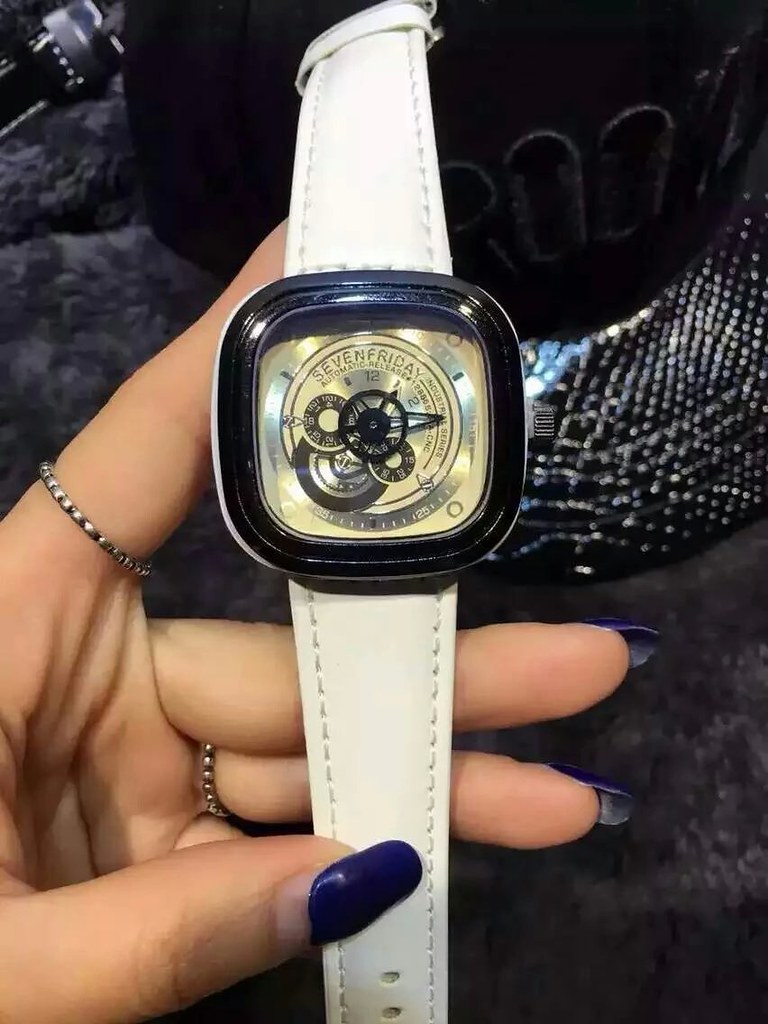This detailed image captures a woman of apparent Caucasian descent, identifiable by her fair skin tone. She is showcasing her meticulously manicured nails, painted in a striking blue color. Adorning her fingers are two elegant rings: one graces her index finger, while the other embellishes her ring finger. The focal point of the image is the sophisticated white leather strap watch that she holds delicately. The watch boasts a captivating black face, intricately designed with visible cogs, numbers, and other mechanical features, indicative of the high-quality craftsmanship associated with the Seven Friday brand. In the background, she holds a stylish bag that adds an extra touch of elegance to the overall composition.